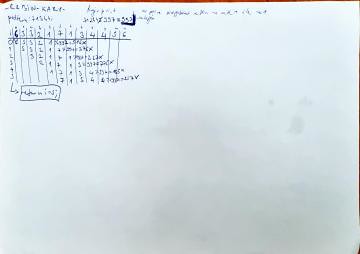An overhead photograph captures a white piece of paper laying on a brown wooden desk. The paper features small, intricate writing primarily located in the top left corner. The writing is divided into sections, some of which are also centered at the very top of the page. The bottom half and the entire right side of the paper remain blank, emphasizing the concentration of details in the upper left quadrant.

The writing and drawings appear to form a type of scoreboard grid. The grid has a horizontal line at the top with numbers above it, segmented by vertical lines. At the bottom left of this grid, an arrow points toward a hand-drawn rectangle containing additional text. All markings on the paper are done with an ink pen. The edge of the brown wooden desk is visible as a thin border along the top and right sides of the photograph, framing the white paper.